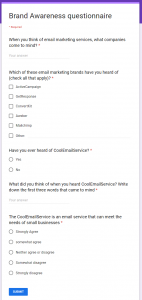The color image depicts a website with a predominantly white background and black text. The top of the page features a narrow purple bar. The image is significantly out of focus, requiring zooming in to over 400% to attempt to read the text, which exacerbates the blurriness and reduces readability. 

The main heading reads "Brand Awareness Questionnaire," followed by a nearly illegible question about categories. Below, there is another question asking about familiarity with email marketing brands, accompanied by a checklist, though the brands are not discernible due to the image quality.

Further down, there is a query involving a word that starts with the letter "C," offering "Yes" or "No" options. The subsequent question prompts for an opinion on an unspecified topic, with space provided for an answer. Lastly, there are five checkboxes with options that can't be read clearly and a blue button at the bottom of the page, which is also out of focus. The overall poor quality of the image severely hinders the ability to interpret its content.